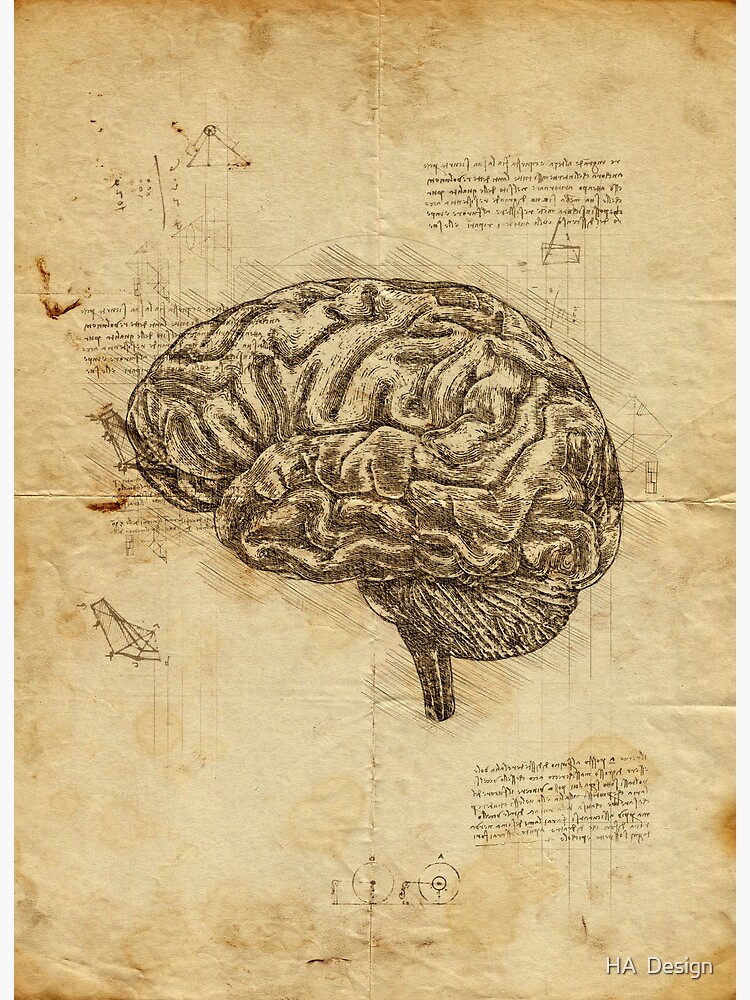The image depicts an aged, yellowing piece of paper with several tan stains and fold marks, reminiscent of an old treasure map. At the center is a highly detailed, black-and-white drawing of a human brain, surrounded by several indistinct pieces of text. Small, barely legible writing is scattered around the brain, specifically in the top left, top right, and bottom right corners of the paper. Additionally, a small drawing of a triangle with a circle atop it is located in the top left of the image. At the bottom, there are two wheels connected by a string system, each with labels over them. In the bottom right corner, the text "H.A. Design" is visible in white with a black border, indicating a watermark or logo. The overall impression is that of a scientific document rather than a piece of artistic artwork.